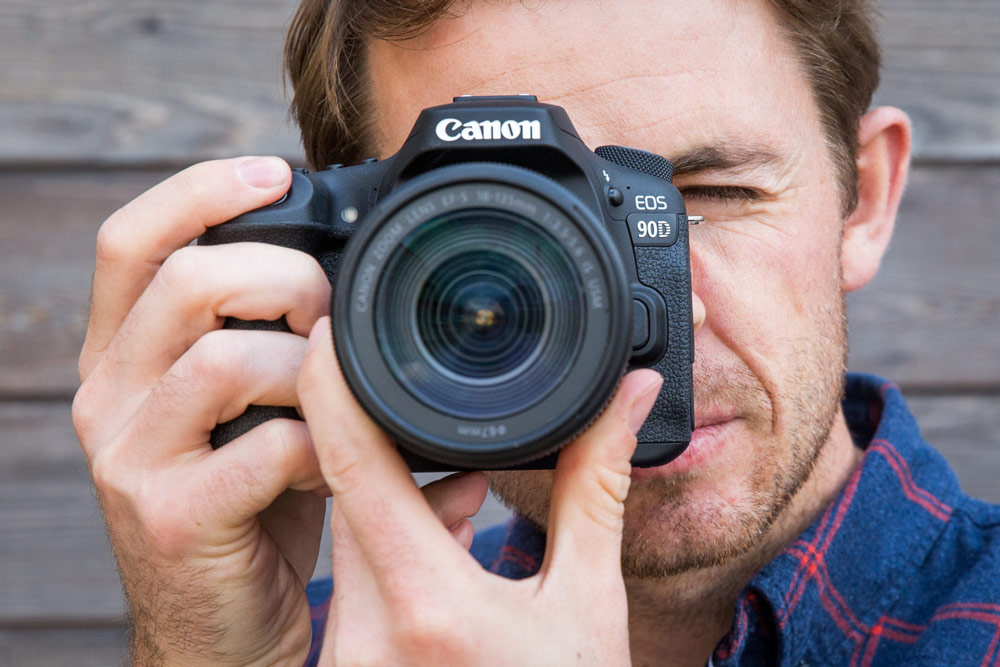In this close-up headshot, a middle-aged, Caucasian man with short, light brown hair and a stubbly beard is seen taking a picture with a Canon EOS 90D camera. The camera's black body features a wide 100 millimeter lens prominently labeled with "Canon". His left hand is positioned around the bottom of the lens, adjusting it, while his right hand holds the camera with his index finger on the shutter button. The man's left eye is focused through the viewfinder, his right eye closed in concentration. He is wearing a blue, flannel-style shirt with red and black stripes and stands against a background of overlapping gray wooden slats.